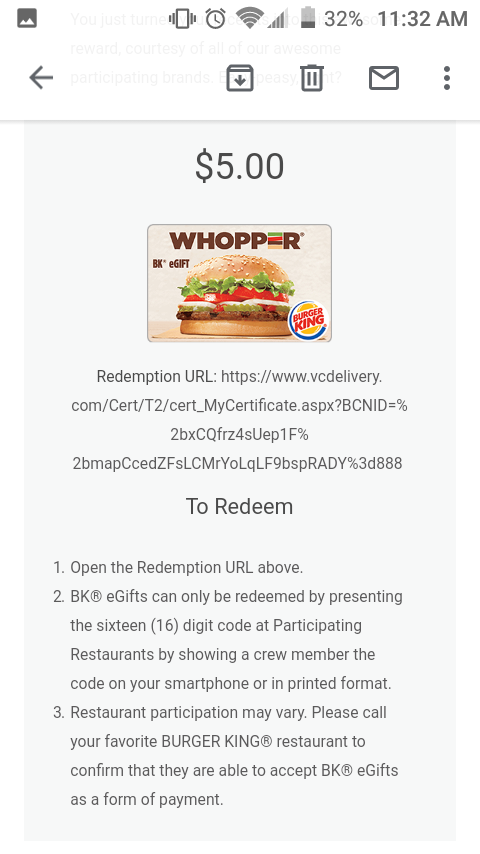This image is a screenshot from an Android mobile device, showcasing various elements from the status bar down to the detailed content of an email. It is 11:32 a.m. as indicated in the top status bar, and the device has 32% battery life. The user has full cell reception with four bars and is connected to Wi-Fi, also showing four bars. The icons suggest that an alarm is set, the device is in silent mode, and a screenshot has recently been taken, as denoted by the screenshot icon in the upper left-hand corner.

The screenshot captures the Gmail app interface. The header of the app features a left-pointing arrow for navigation, a trashcan icon for deletion, an envelope icon, and a three-dot menu for additional options. The background of the app is predominantly light, with the email content contrasting against a slightly lighter gray background.

The email itself is an offer from Burger King. The header of the email prominently displays "$5" in black text, followed by an enticing image of a Whopper. Adjacent to the image is the Burger King logo positioned in the bottom right-hand corner. The email includes a "redemption URL," represented by a lengthy website link intended for the user to copy and paste into their browser. Following the URL, the email provides instructions for redeeming a $5 gift certificate to Burger King, outlined in three steps.